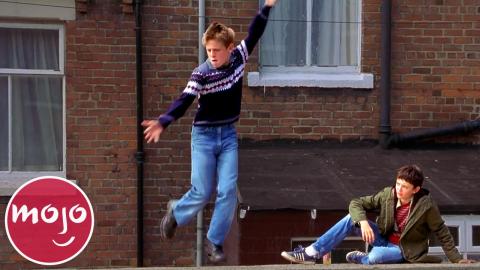This image, reminiscent of a scene from a vintage movie, captures two young boys against the backdrop of a red brick building. The boy mid-air, striking a diagonal pose with one arm raised high and the other lowered, is the spitting image of a young Kevin Bacon from "Footloose." He sports a classic 1970s winter sweater adorned with snowflakes at the top, blue jeans, and black shoes, his short blonde hair catching the light. Beside him, another boy sits on the ground, dressed in an olive-green jacket and blue jeans, observing the spirited leap. In the lower left corner, there's a distinctive logo for Mojo—a circle with a white border, the word "Mojo" stylized to resemble a face with a smiley mouth below. The scene is undeniably set outdoors, possibly showing a dumpster or shed in the background.